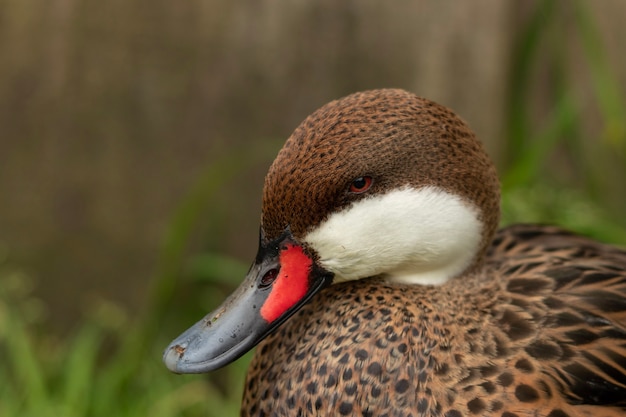This image captures a close-up of what appears to be a young duck or duckling, focusing on the delicate features of its face and head. The duckling's head is predominantly dark brown, topped with darker feathers that could be described as almost greenish-brown in some areas. A striking feature is a large red marking near its eye, which is closed into a slit, giving the bird a peaceful or resting appearance. The top of its head transitions into a bright white area below its eye, extending to the neck, which is adorned with tan feathers speckled with darker brown or black spots. The beak is predominantly dark brown, accented with a red stripe near the base. The background is a soft blur of green grass and trees, allowing the duckling's detailed and textured plumage to remain the focal point of the image. The picture provides an intimate and tender glimpse of this small creature, emphasizing the patterns and colors of its feathers against a natural, though slightly out-of-focus, backdrop.